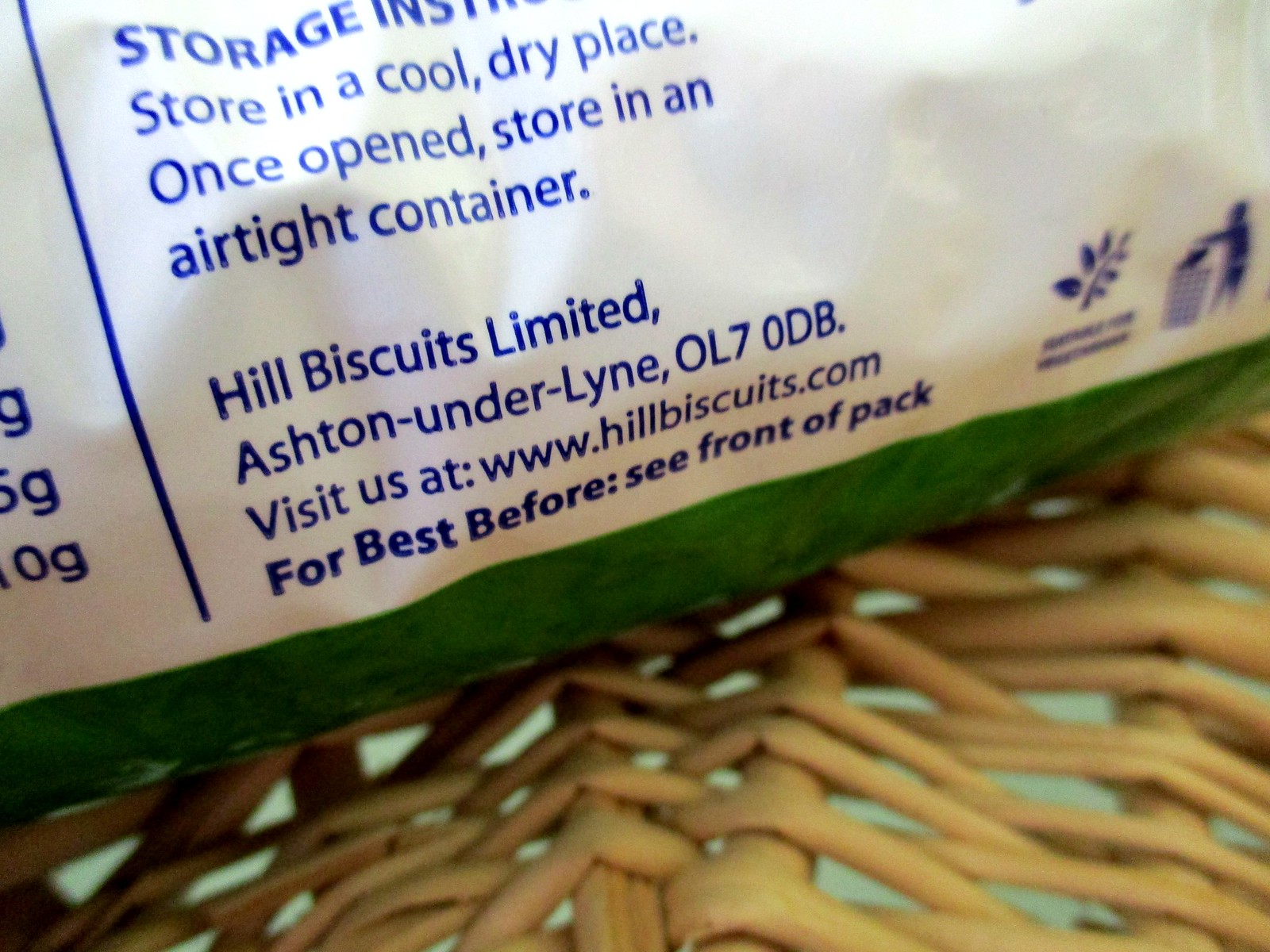The image depicts the bottom portion of a white plastic bag with blue lettering and a green trim, resting on a light beige woven wicker surface that only takes up the bottom part of the picture. The bag's blue text prominently displays "STORAGE" in all caps, followed by instructions: "STORE IN A COOL, DRY PLACE. ONCE OPENED, STORE IN AN AIRTIGHT CONTAINER." Below this, the bag is marked with "HILL BISCUITS LIMITED, ASHTON-UNDER-LYNE OL7 0DB," and a web address: "WWW.HILLBISCUITS.COM." Further down, it advises, "FOR BEST BEFORE, SEE FRONT OF PACK." The right side of the bag features blue printed illustrations, including a stem with leaves and a figure throwing something into a trash bin, suggesting recycling.